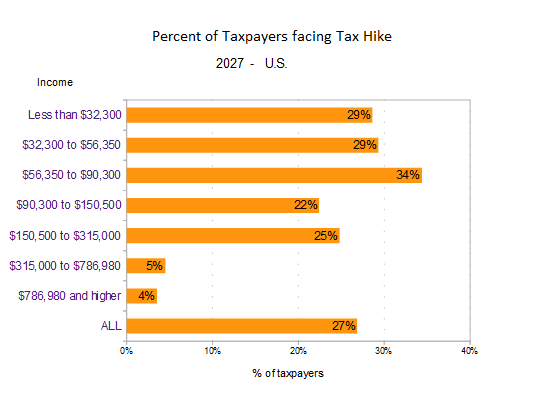The image is a detailed horizontal bar chart set against a white background, titled in black text as "Percent of Taxpayers Facing Tax Hike 2027 - US." Below the title, the x-axis is labeled "Percent of Taxpayers," with increments ranging from 0% to 40% in 10% steps. The y-axis, shaded in blue, is labeled "Income" at the top and lists income brackets as follows: "All," "786,980 and higher," "315,000 to 786,980," "150,500 to 315,000," "90,300 to 150,500," "56,350 to 90,300," "32,300 to 56,350," and "Less than 32,300." Orange bars extend horizontally across the chart, representing the percentage of taxpayers facing a tax hike in each income bracket, with percentages printed in black on these bars. The largest bar, corresponding to the income bracket "$56,350 to $90,300," displays "34%." Other notable percentages include "29%" for both "Less than $32,300" and "$32,300 to $56,350," "22%" for "$90,300 to $150,500," "25%" for "$150,500 to $315,000," "5%" for "$315,000 to $786,980," and "4%" for "786,980 and higher." The "All" category shows "27%."